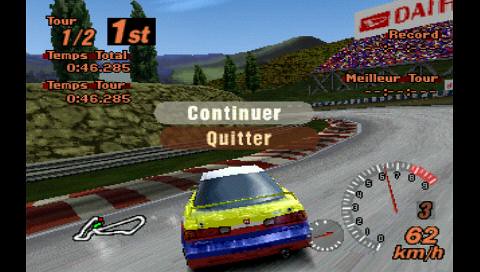In this detailed screenshot from a pixelated video game racing scene, we see a sedan-type vehicle navigating a mid-turn on a road course. The vehicle's top half is white transitioning to yellow, followed by a blue stripe and a black bumper with hints of red around it. This car, central to the image, is paused as indicated by the "CONTINUER" and "QUITTER" options in the middle of the screen, suggesting a French language setting.

In the top right corner, the text "RECORD" and "Miur Tour" is visible, while the top left corner displays "Tour 1 out of 2," indicating the first lap of the race. The racer is currently in first place. In the lower right corner, a speedometer ranging from 0 to 9, with a hint of red, shows the car's speed at zero with "62 KM/H" next to it. At the bottom left, there's an icon representing the current course layout. The overall pixelated graphics reinforce the video game environment.